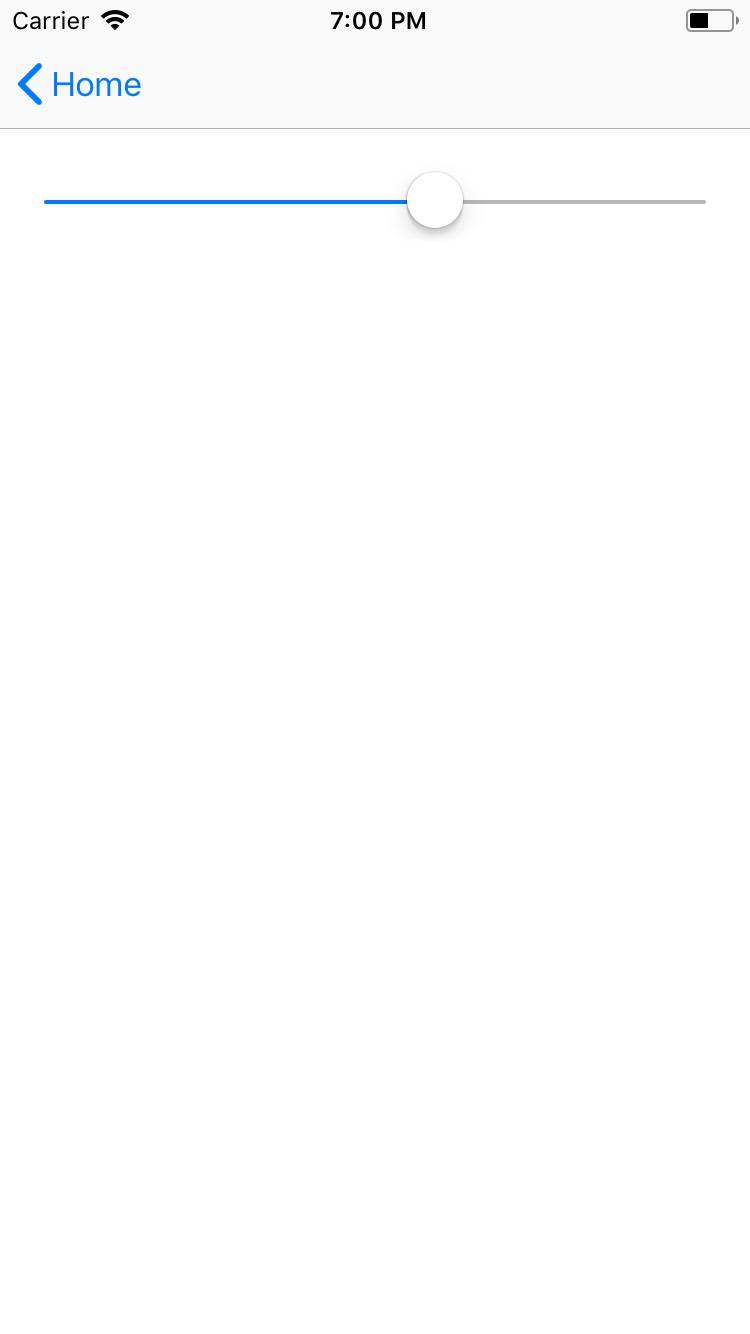The image presents a simplistic, almost minimalist, depiction of a user interface element commonly seen on mobile devices. The layout is within a horizontally oriented rectangle, which mimics the top bar of a smartphone screen. 

At the top-left corner, the word "Carrier" appears, likely as a placeholder text, accompanied by an icon representing signal strength, depicted as three expanding bars forming a pie shape. Centrally positioned is the time display, reading "7 p.m." On the top-right corner, a battery icon signifies the battery status.

Further down, in the bottom left corner of this rectangle, there is a blue left-pointing caret arrow, labeled "home" in blue text, indicating a navigational button that can be tapped to return to the home screen.

Beneath this top bar, there's a centrally justified horizontal slider occupying approximately 85% of the width of the rectangle. The slider features a movable white circle, which currently rests approximately two-thirds of the way along the slider. The leftmost two-thirds of the slider are filled in blue, suggesting that the user has adjusted this control to two-thirds of its maximum potential, while the remaining rightmost portion remains gray, indicating unselected space.

The entire composition is rendered in a clean, black font with subtle blue accents, indicative of a streamlined user interface likely intended for a digital prototype or UI/UX design mockup.